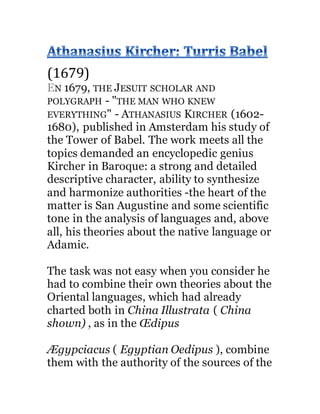The image is a screenshot of text from an internet source, featuring a detailed description of Athanasius Kircher's 1679 work, "Turris Babel." In black and blue lettering, the text begins with the title "Athanasius Kircher, Turris Babel," followed by "1679." The main body of the text notes that in 1679, the Jesuit scholar and polygraph, often referred to as "the man who knew everything," published his study of the Tower of Babel in Amsterdam. The description emphasizes Kircher's encyclopedic genius, noting his ability to synthesize and harmonize authorities with strong and detailed descriptive character. The heart of his work is influenced by Saint Augustine, containing a scientific tone in the analysis of languages, particularly his theories about the native or Adamic language. The task of producing this work was notably challenging as Kircher had to integrate his theories about Oriental languages, previously charted in "China Illustrata" and "Oedipus." The text continues beyond this summary.